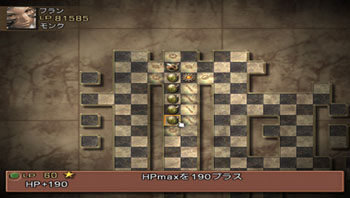This rectangular photo captures a screenshot of a strategic video game reminiscent of chess, but with a unique twist. The game board is irregular, featuring missing tiles and round game pieces instead of the traditional square ones. The background is a faint tan, tile-like pattern, adding texture without overpowering the scene. Chinese characters are subtly overlaid, indicating potential in-game elements or settings.

Prominently displayed at the bottom of the screen is a large red bar labeled "HP," showing a current value of 190 with some yellow numbers preceding it. In the center of this bar, a label reads "HP MAX," followed by additional numerical values. In the top-left corner of the screen, there is a small box containing an avatar's face, accompanied by a series of numbers.